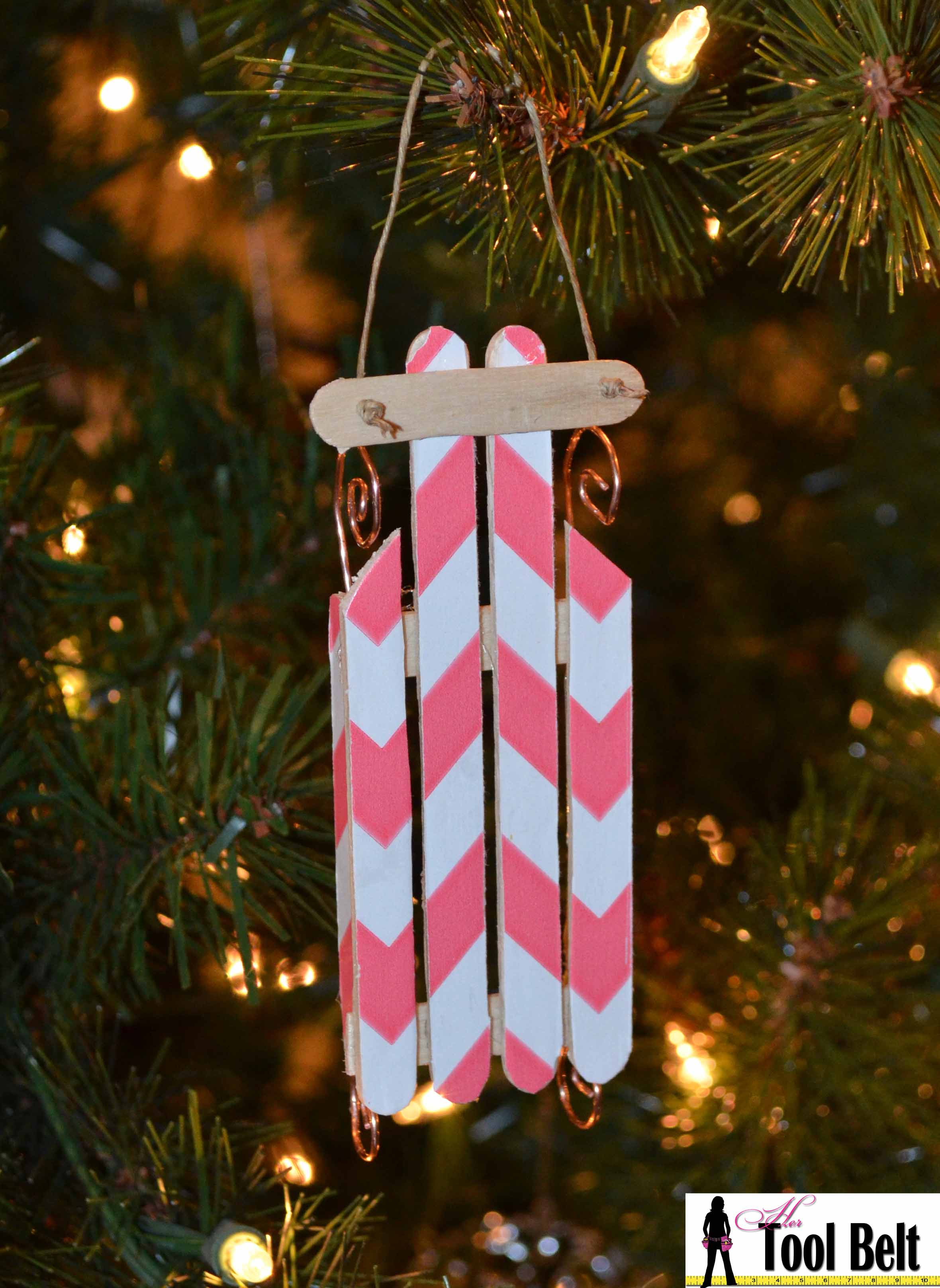This close-up photograph captures a charming, homemade Christmas ornament hanging from a branch of an artificial Christmas tree adorned with white, yellow, green, and orange lights. The ornament is a miniature sled crafted from painted Popsicle sticks, arranged in a chevron pattern of red and white diagonal stripes. The sled features intricate copper wire runners curving gracefully at the top and bottom edges. In the lower right-hand corner of the image, there is a logo of a silhouette of a woman with a tool belt beside the text "Her Tool Belt," lending a personal and handcrafted feel to the scene.